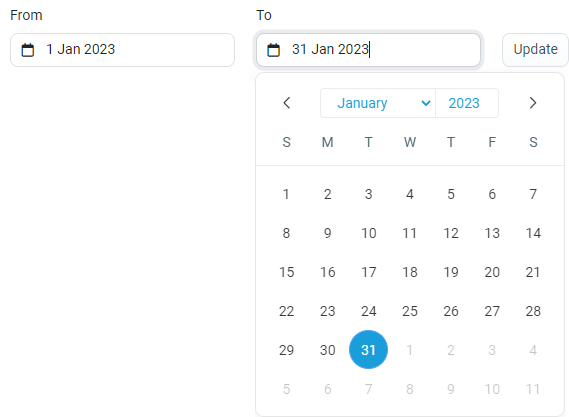The image is a high-quality, unblurred screen capture featuring a calendar interface set on a white background. On the left side of the image, there is text in black font that reads "From", followed by a gray box containing a small black calendar icon and the date "1 Jan 2023". On the right side, it says "To", followed by another gray box with a similar black calendar icon and the date "31 Jan 2023". Below this is another gray box labeled "Update" in gray text.

Beneath this section, the main calendar for January 2023 is depicted. It includes a black "back" arrow, two blue dropdown boxes—with the first labeled "January" and a corresponding blue pull-down arrow, and the second labeled "2023". Another black arrow is present next to these dropdowns, likely for navigation.

The calendar itself displays the days of the week from Sunday through Saturday at the top, followed by the individual days of January. The 31st of January is specifically highlighted with a blue circle, and the date "31" is in white. The rest of the days are shown in a blackish-gray color. Additionally, the calendar extends into February, showing dates from the 1st through the 11th of the following month.

Overall, the screen capture is noted for its excellent visual quality, with no pixelation or blurring, making it very user-friendly for low vision users. There are no other images or elements to describe, ensuring a clear and focused visual experience.